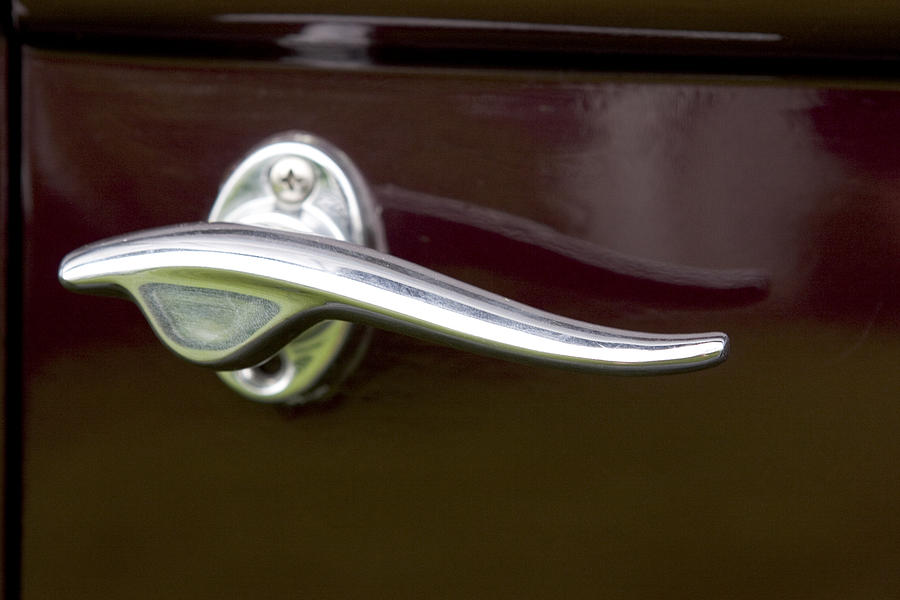The image depicts a close-up of a vintage, chrome door handle, possibly from an antique car, mounted on a deep reddish-maroon surface. The handle, which pivots and features a long, shallow curve, brings to mind a porpoise gliding through water. The metallic surface reflects the handle, enhancing its sleek, streamlined appearance. A chrome bolt secures the handle, and a black accent, likely the lining of a window, is visible in the background. The overall aesthetic has a soft, diffused quality, giving the impression of a painting or a purposefully blurry photograph, evoking the classic cars of the 1940s or 1950s.